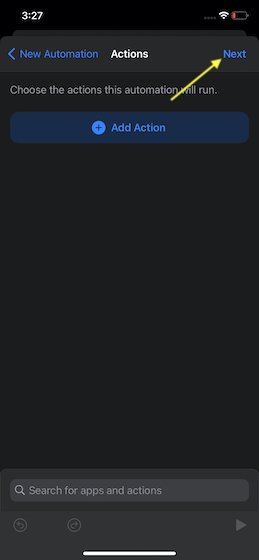This is a screenshot from a smartphone displaying an app interface against a dark black background. In the top left corner, the time is shown as "3:27". On the far right of the top edge, a Wi-Fi signal icon, depicted as a "V" with four fully filled bars, indicates strong connectivity. Next to the Wi-Fi signal, a battery icon with a grey outline and a thin red bar at the bottom illustrates a low battery level.

Below the top status indicators, there is a dark gray bar with blue text and a left arrow. From left to right, the centered text reads, "New Automation" in white letters, flanked by the word "Actions" on the left and "Next" in blue letters on the right. 

Underneath this bar, a light gray text reads, "Choose the actions this automation will run," aligned to the left over a black background. Directly beneath this text, there is a dark blue rectangular bar featuring a bright blue dot with a black plus symbol in its center, followed by the phrase "Add Action" in blue letters.

Superimposed over the middle of the screen is a yellow diagonal arrow pointing from the "Add Action" button towards the "Next" button. 

At the very bottom of the screen, a grayed-out search field displays the placeholder text, "Search for apps and actions".